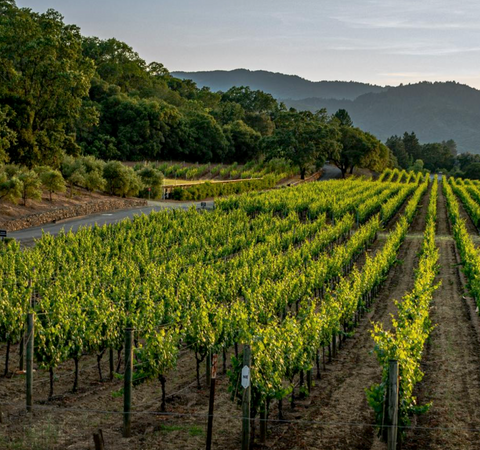This photograph captures a picturesque agricultural scene in a sprawling vineyard that extends across multiple fields. The vineyard is meticulously arranged in symmetrical rows of young, vibrant green sapling trees with shades ranging from the lightest lime to the deepest forest green. The earth between the rows varies from dark, rich soil to autumnal browns, perfectly contrasting the lush foliage.

In the background, the vineyard is bordered by densely leafed dark green bushes and trees, which gradually transition into a mountainous region to the back right of the image. These mountains, cloaked in a bluish hue and dotted with more trees, create a serene and expansive backdrop. To the top left, a cluster of dark green trees adds depth to the landscape.

The sky above is a pale white, possibly indicating an overcast day or the soft light of dusk. A road runs alongside the vineyard, guiding the eye through this well-maintained pastoral setting. The meticulous rows of vegetation demonstrate a well-planned monoculture, where each sapling, with its bright green leaves and occasional yellow highlights from flowers, thrives in its neatly plowed patch of earth. This idyllic scene exemplifies the beauty of a well-tended vineyard amidst a natural, mountainous landscape.